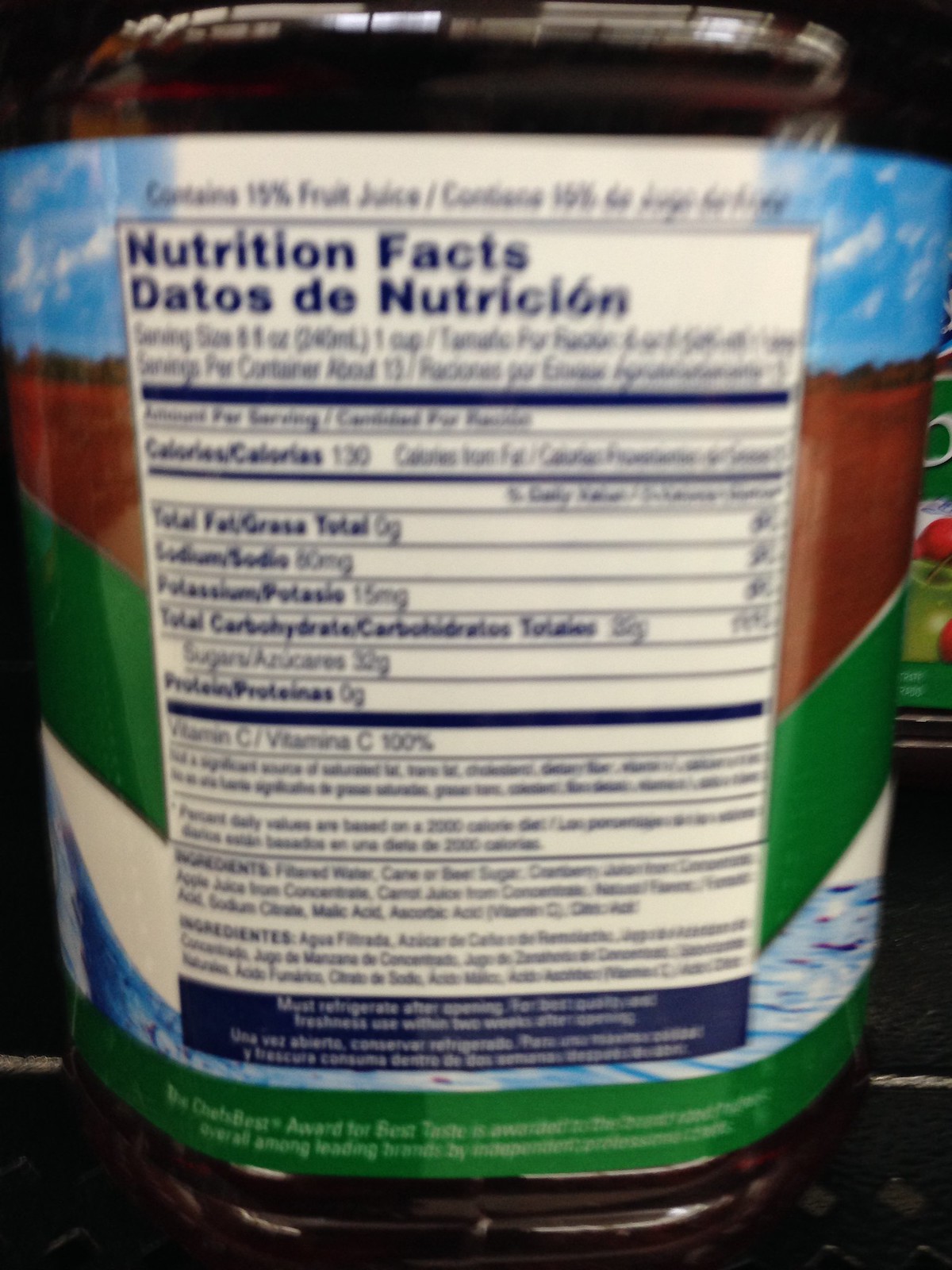This image is a close-up of the back of a fruit juice container, specifically the nutrition facts label. The photo is slightly blurred, making some details difficult to read. At the top, it states in both English and Spanish, "Contains 15% fruit juice." Below that is more text which is blurred and unreadable. The label features a white box with blue writing, stating "Nutrition Facts" and "Datos de Nutrición." The serving size is listed as six fluid ounces, one cup. The calorie count is 130, although the "calories from fat" text is blurred. The label lists total fat as zero grams, sodium as 60 milligrams, potassium as 15 milligrams, total carbohydrates and sugars both as 32 grams, protein as zero grams, and vitamin C as 100 percent.

The design includes multiple colored stripes: a dark green stripe, a chocolate brown stripe, a white stripe, and a cyan blue stripe, running vertically along the label. The juice container's label begins with a blue sky section at the top, followed by brown, green, and white sections that include blue water patterns, descending down towards more green at the bottom. The container is resting on a table. This description suggests it could be a cranberry juice by Ocean Spray.